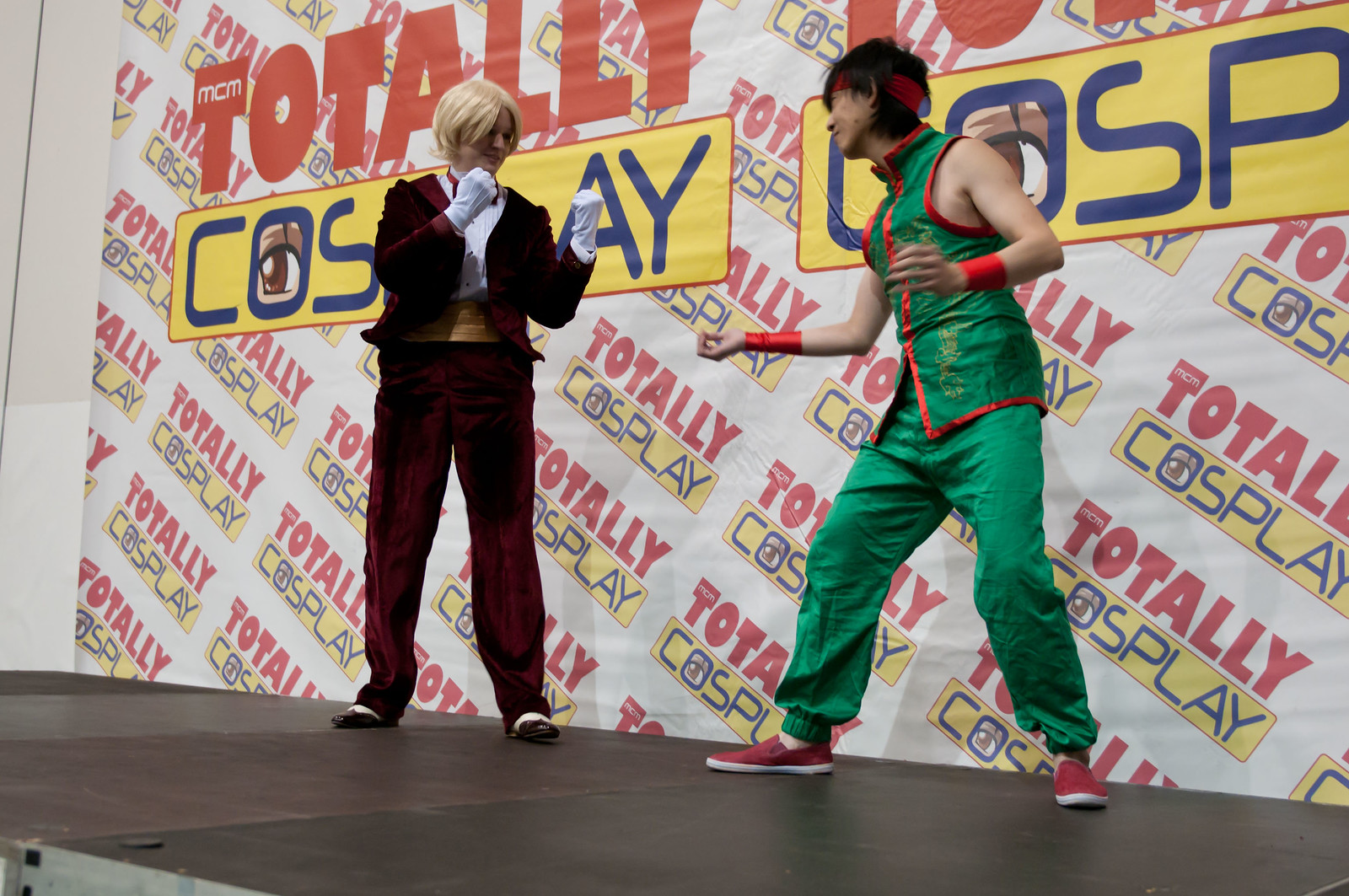In this photograph, two people are captured on stage in elaborate costumes, with the backdrop marked with the words "Total Cosplay." On the right, a man is striking a karate pose, dressed in a sleeveless green outfit complemented by a red bandana, red wrist wraps, and red sneakers. On the left, the person, possibly wearing a short blonde wig, is dressed in an elaborate, dark brown velvet suit with a yellow-gold cummerbund, a white shirt, and white gloves. This individual has their arms raised and is making fists, adding to the dynamic energy of the scene.